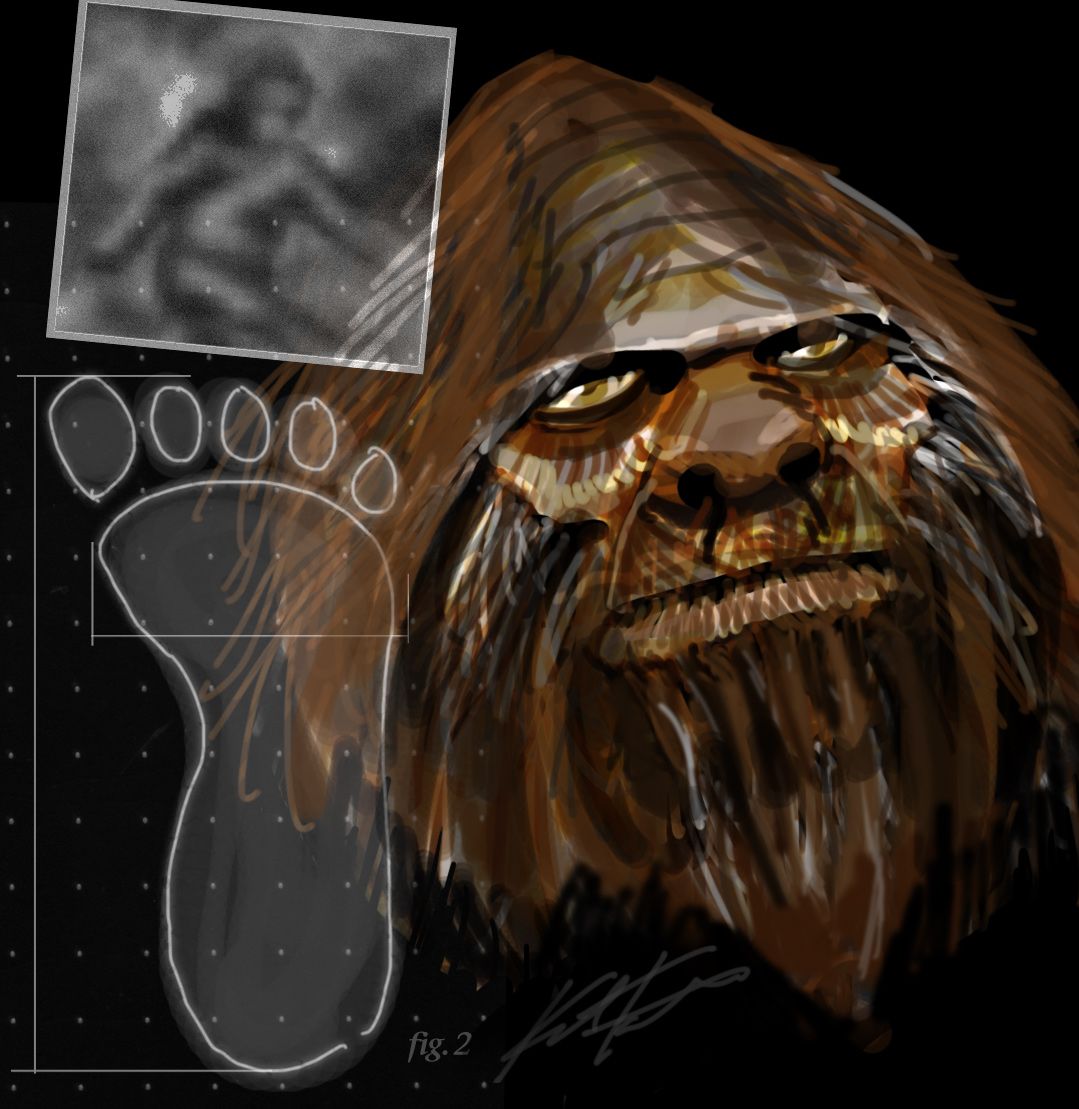The image features an artistic representation of Bigfoot's head, characterized by a pointed top, overhanging brow, scraggly hair, and a beard. Bigfoot's head is depicted in shades of brown, black, and tan, set against a black square background. On the upper left corner, there is a square, black-and-white blurry image capturing a humanoid figure's torso, head, and upper legs, reminiscent of the iconic Bigfoot footage. The left-hand side also features a large transparent footprint outline, drawn in white on a gray background, depicting a foot with a prominent big toe and four other toes. Bigfoot's head partially overlaps these two transparent elements, blending them into the composition and giving the entire piece a layered depth.